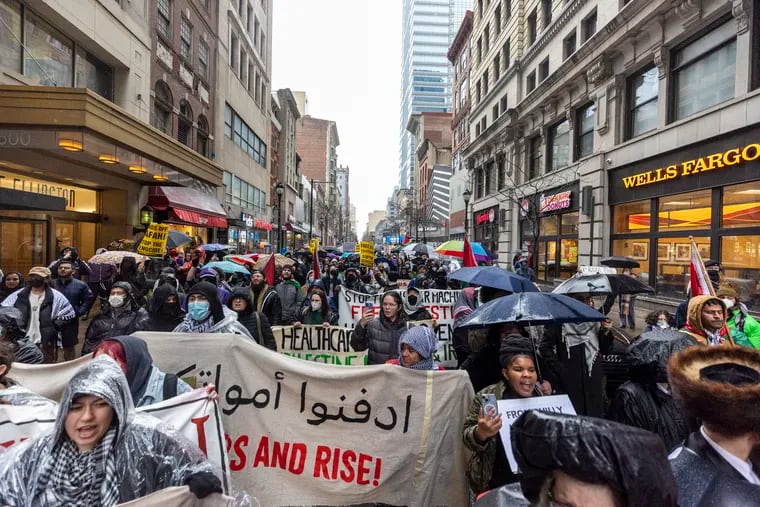This outdoor daytime photograph captures a bustling protest on a narrow city street in downtown New York. Flanked by rows of buildings, including recognizable storefronts like Wells Fargo on the upper right and Dunkin' Donuts on the left, the street is densely packed with protesters of diverse ethnic backgrounds. Amidst the crowd, umbrellas and raincoats indicate a rainy day, while some attendees also wear face masks. The sky above is a muted white, contributing to the overcast atmosphere.

Protesters fill the entire street, holding a variety of signs and flags, some with messages addressing health care and others displaying text in different languages, including Arabic. Partial slogans suggest themes like "health care," "Palestine," and "rise." Dotted with shades of red, orange, yellow, green, gray, black, white, aqua blue, and beige, the scene etches a colorful, powerful image of civic engagement against the backdrop of towering city structures.